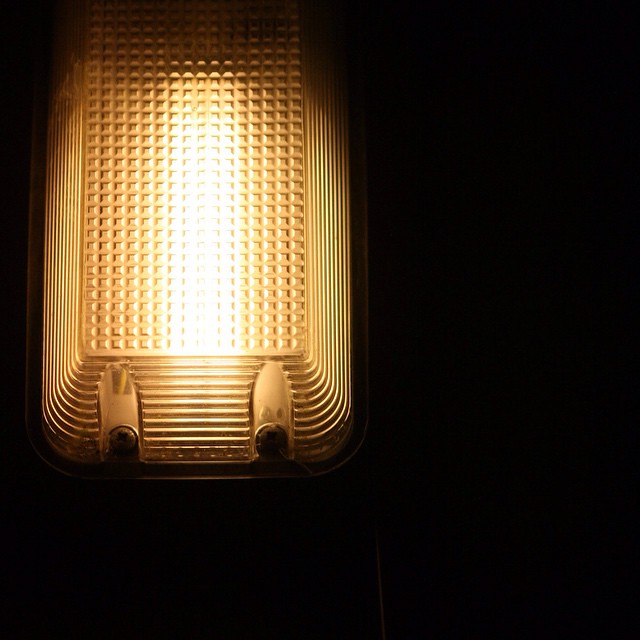This photograph features an illuminated lamp or lantern set against a completely black background, creating a striking contrast. The lamp, potentially an outdoor light or sconce, emits a bright white light from within, highlighting its intricate design. The front of the lamp is rectangular, adorned with a unique basket weave pattern comprised of tiny squares on its surface. Surrounding the light are several lines, adding to its textured appearance, while the sides show rectangular steps that gradually elevate to support the structure. The lamp cover, likely made of a plastic material, is notably secured with two screws, showcasing both functionality and design. Additionally, in the upper left corner of the image, there's a distinct golden, rectangle-shaped object that enhances the visual interest of the scene.